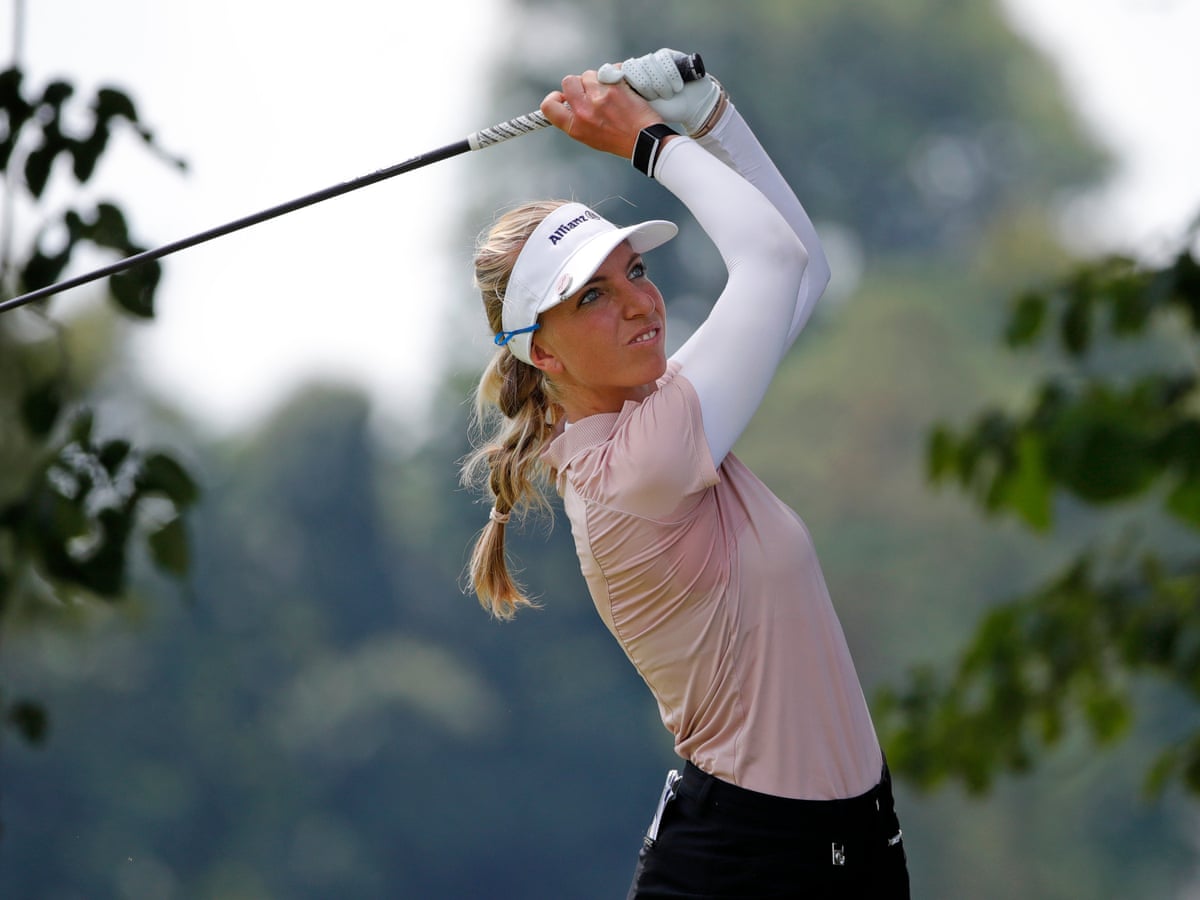The image showcases a female golfer, centrally positioned, in the midst of completing a swing with her club held behind her head. She is outfitted in a light pink shirt layered over a white long-sleeve top, with both her arms covered in white cloth. She wears a white visor emblazoned with the word "Allianz" in blue, paired with black pants. Her long blonde hair is neatly tied back into a ponytail. On her right hand, a smartwatch is visible, and both hands are gloved in white, firmly gripping a black club. The background, though very blurry, features patches of green foliage and hints of larger trees against a gray sky, indicating a daytime setting.